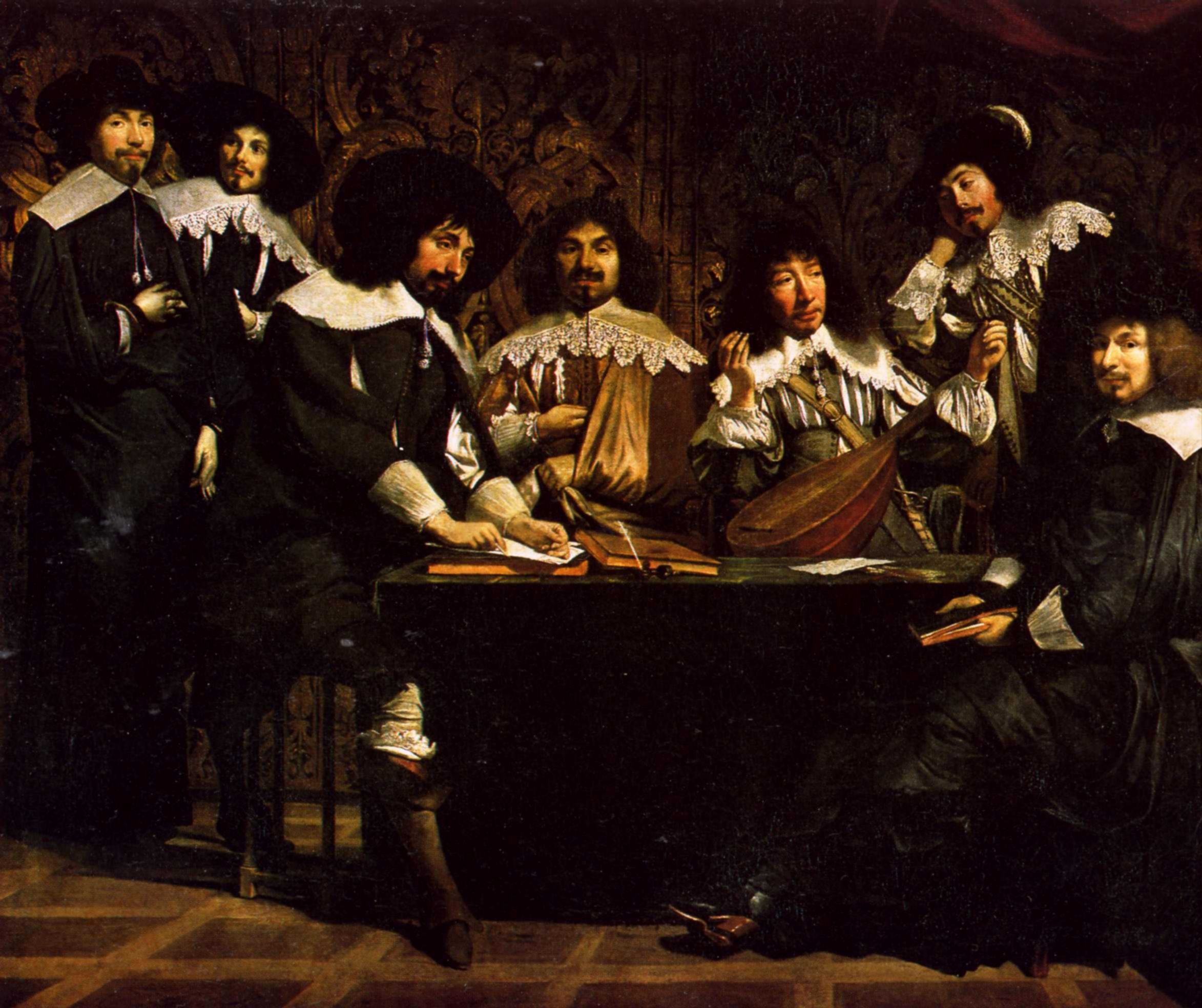This is a wide rectangular painting in an old, almost Renaissance style, depicting a group of seven men gathered around a black, rectangular table that starts at the right middle side and extends inward, stopping just past the center. The floor consists of dark brown tiles separated by a lighter brown material. The men are dressed in old-fashioned, upper-class outfits with elaborate, frilly collars and poofy, long black sleeves, indicative of a wealthy Victorian or Renaissance lifestyle. Each man has similar facial features, sporting mustaches and goatees, and shoulder-length, bushy black hair that gives them a familial resemblance. 

To the right, a man in all black with a white collar sits in front of the table with his legs crossed. Behind the table, three men in fancy attire hold musical instruments. The table itself features several brown and orange books, suggesting scholarly or musical activities. On the left side, two men stand side-by-side, wearing large black hats and ornate clothing, gazing outward as if looking at the viewer. The setting appears to be a dark room with ornate wallpaper, reinforcing the old-fashioned, upper-class ambiance.